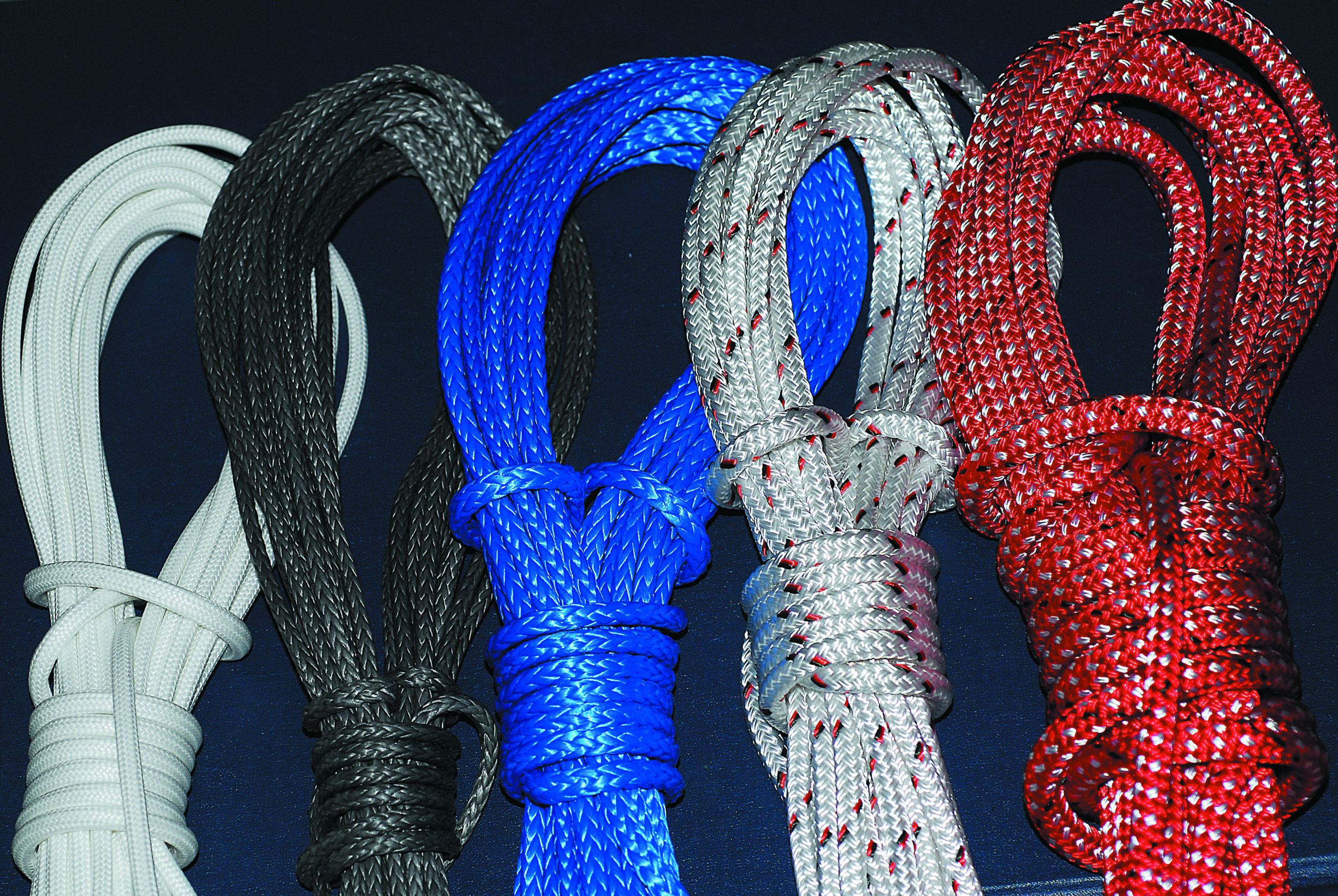This color photograph in landscape orientation showcases five distinct bundles of coiled, twisted nylon ropes, arranged side by side against a stark black background. Each bundle is meticulously tied at the center, creating loops at the top, secured by multiple wraps of the same rope. From left to right, the ropes display a vivid spectrum: the first bundle is solid white, followed by a solid black rope, then a vibrant royal blue. Next to them is a white rope intricately speckled with red flecks, and the sequence culminates with a striking red rope dashed with white and black flecks. These ropes, known for their durability and resistance to fraying, are reminiscent of versatile nylon ropes commonly employed in various practical applications. The photograph, captured in a style that emphasizes Photographic Representationalism and Realism, gives a detailed and true-to-life representation of these essential, multi-colored nylon ropes, highlighting their texture and robust utility.